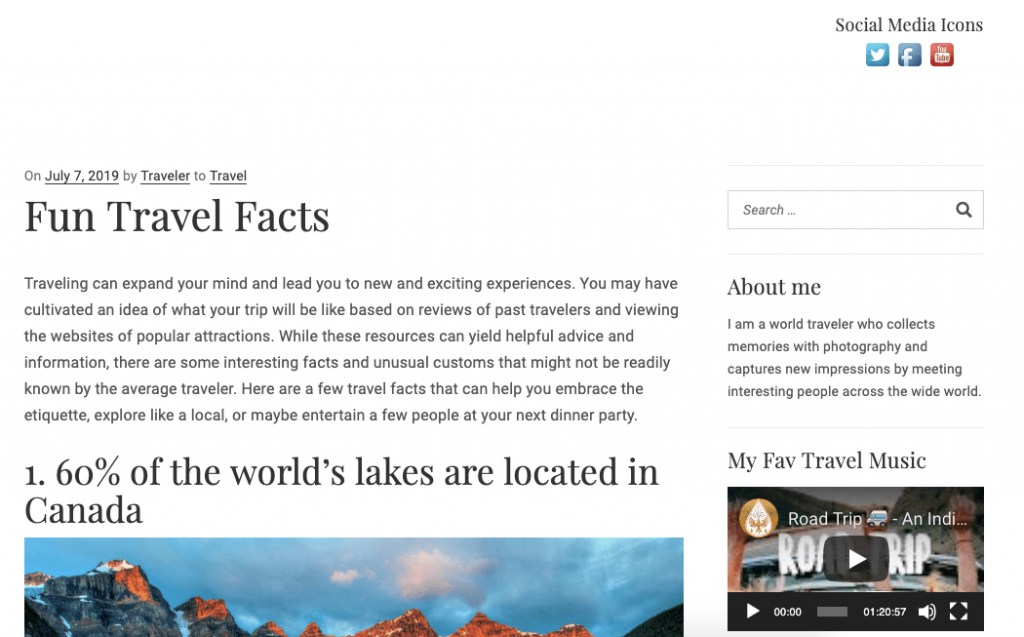A webpage from a travel blog featuring an article titled "Fun Travel Facts," posted on July 7th, 2019, by Traveler to Travel. The site has a CNN-like appearance, with social media icons for Twitter, Facebook, and YouTube at the top right, and a search bar just below them. The "About Me" section highlights the blogger as a world traveler who captures memories through photography and connects with interesting people globally. The article suggests that while travel resources provide helpful advice, they may overlook fascinating facts and unique customs. The first fact listed is that 60% of the world's lakes are located in Canada, accompanied by a serene image of a lake.